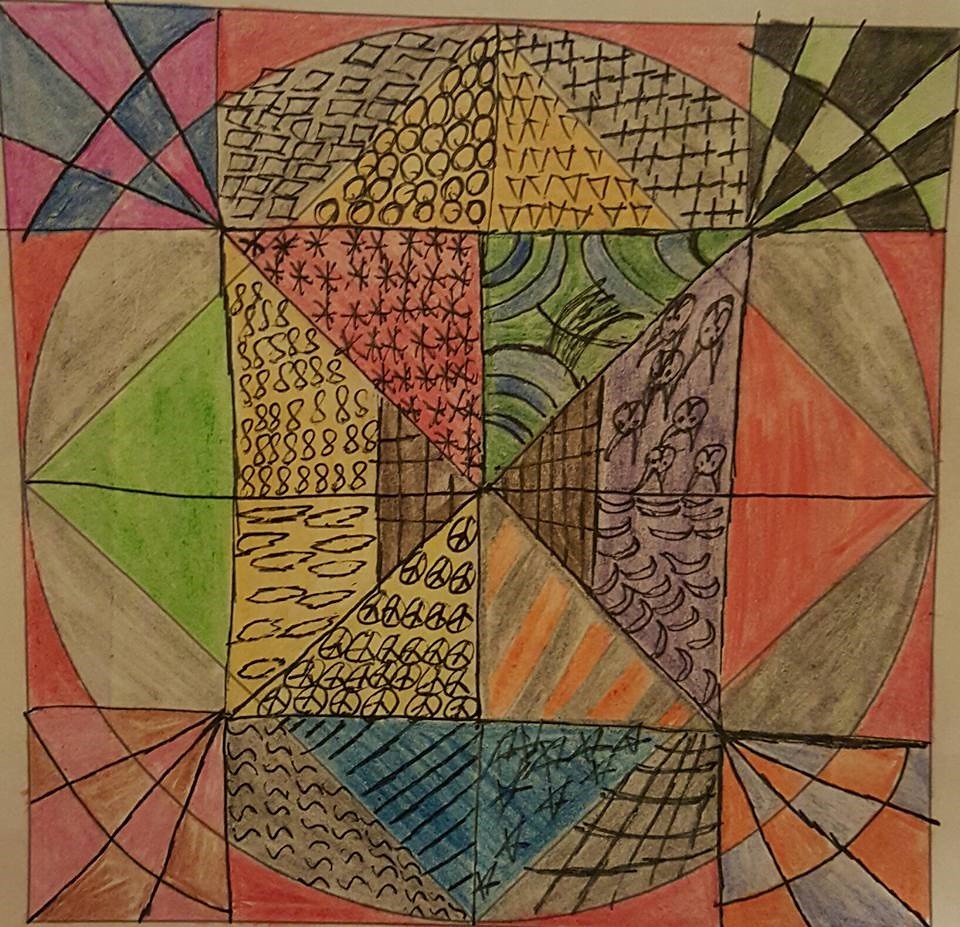This intricate artwork is a drawing created with an ink pen and vividly colored using colored pencils. The design resembles a quilt pattern, showcasing a harmonious blend of geometric precision and vibrant hues. The layout consists of a grid with four squares across the top, four squares down each side, and a central section composed of four squares, each subdivided into two triangles.

The corner squares are meticulously patterned with alternating checks in captivating color combinations: pink and blue, brown and green, orange and purple, and pink and brown. The central area presents a more complex arrangement, with each square within the middle section divided into two triangles. These triangles are carefully placed to form a dynamic interplay of shapes, creating a visual symphony that draws the viewer's eye across the entire piece. The thoughtful use of colors and patterns gives the artwork a sense of depth and unity, making it a compelling and mesmerizing composition.